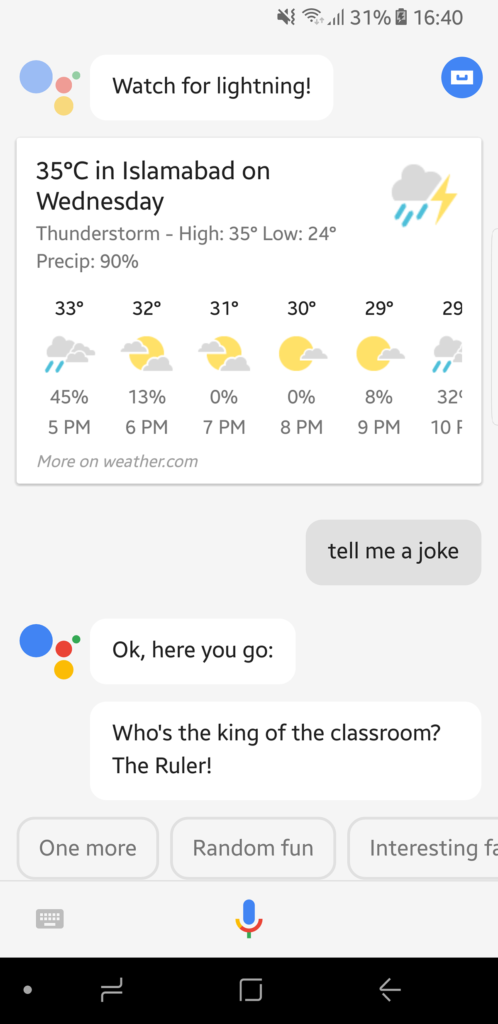**Detailed Descriptive Caption for an Image of a Smartphone Interface:**

The image is a screenshot of a smartphone interface displaying the Google virtual assistant application. Prominently featured at the top is a weather update for Islamabad. The main forecast for Wednesday indicates a high temperature of 35 degrees Celsius with a low of 24 degrees Celsius. A thunderstorm is expected, with a graphic icon depicting a cloud, rain, and lightning bolt, signifying thunderstorm conditions. The chance of precipitation is 90%. 

Below the main forecast, there's an hourly breakdown for the evening from 5 PM to 10 PM showing changing weather conditions and temperatures:

- **5 PM:** 33 degrees Celsius, 45% precipitation, cloudy with rain.
- **6 PM:** 32 degrees Celsius, 13% precipitation, partly cloudy.
- **7 PM:** 31 degrees Celsius, 0% precipitation, clear.
- **8 PM:** 30 degrees Celsius, 0% precipitation, clear.
- **9 PM:** 29 degrees Celsius, 8% precipitation, partly cloudy.
- **10 PM:** 29 degrees Celsius, 0% precipitation, cloudy with rain.

At the top of the screen, a notification indicates a watch for lightning.

Below the weather update, the user has typed a request, "Tell me a joke." The virtual assistant responds with, "Okay, here you go. Who is the king of the classroom? The ruler." Immediately below the joke, there are three interactive suggestion buttons labeled "One More," "Random Fun," and "Interesting Facts" for further engagement.

The interface also shows that the smartphone battery is at 31%, and the current time is 16:40. The virtual assistant's response area features colorful icons consistent with Google's branding. At the bottom of the screen, a microphone icon is present, indicating the option for voice input.